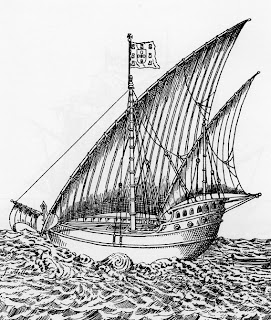The image is a detailed black-and-white line drawing, potentially a woodcut, of an old-time sailing ship, reminiscent of the 17th to 19th centuries. It features intricate line shading and some crosshatching, predominantly around the back of the boat. The ship, likely resembling a schooner or Spanish galleon, is depicted with two sails and one mast, adorned with ropes and rigging that keep the sails fully open. At the top of the mast flies a flag featuring a shield and indistinguishable details. The vessel's hull includes small, dark windows suggesting a lower deck area. The boat is sailing through choppy, swirling waves, moving towards the left side of the image. No people or animals are visible on or around the boat, and the background is completely white, emphasizing the motion and isolation of the ship on the ocean. A smaller vessel appears to be trailing behind the larger ship.